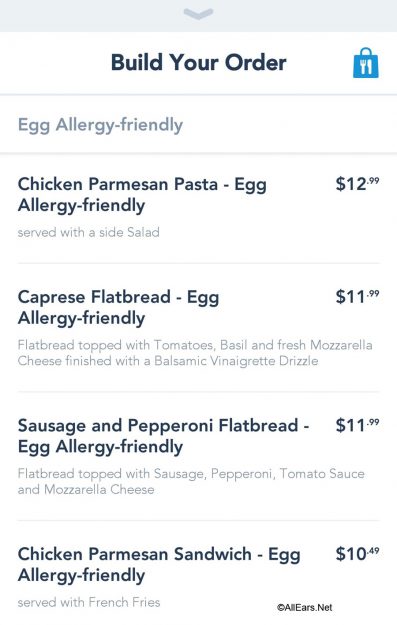The image depicts a computer screen displaying an online menu with a predominantly white background. At the top of the screen, a faint gray rectangle contains a downward-pointing arrow and black text that reads "Build Your Order." To the right of this area is a small, bluish icon resembling a bag, featuring a white fork and knife symbol.

Below the top section, a faint gray line separates the header from the menu items. The first menu item listed is "Chicken Parmesan Pasta - Egg Allergy-Friendly," described as being served with a side salad and priced at $12.99. 

Further down, the next item is "Caprese Flatbread - Egg Allergy-Friendly," which includes a flatbread topped with tomato, basil, and fresh mozzarella cheese, finished with a balsamic vinaigrette drizzle. This item is priced at $11.99. 

Another faint gray line delineates the sections, leading to the next item: "Sausage and Pepperoni Flatbread - Egg Allergy-Friendly." This flatbread is topped with sausage, pepperoni, tomato sauce, and mozzarella cheese, also priced at $11.99.

Finally, another faint gray line precedes the last item: "Chicken Parmesan Sandwich - Egg Allergy-Friendly," which is served with french fries and priced at $10.99 or $10.49.